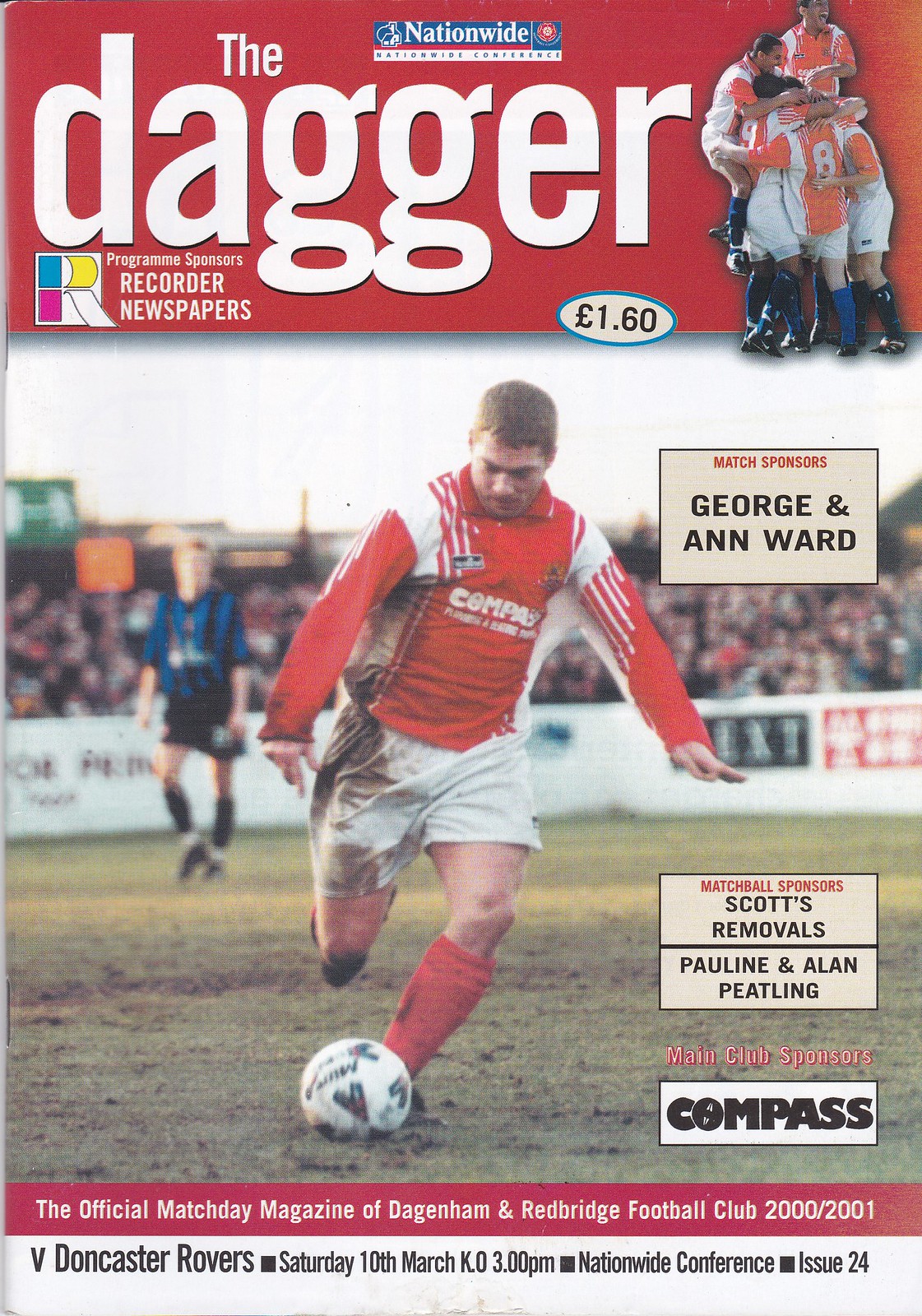The magazine cover prominently features the title "The Dagger" in bold white letters against a red background at the top. Below this, there's the logo of Recorder Newspapers, which comprises a white 'R' within a square filled with blue, pink, and yellow segments. Next to this, the text "Program Sponsors" is visible. A highlighted circle indicates the price as 1.60 Euros.

The central image showcases a soccer player dressed in a red and white striped shirt, white shorts, and red-striped socks, caught in a dynamic moment about to kick a soccer ball. The player is notably covered in dirt, emphasizing the action and roughness of the game. In the background, blurred but noticeable, are spectators behind a white barrier and a referee donned in a blue and black uniform.

Sponsors' names are listed to the right of the central figure within gray boxes, including "George and Ann Ward," "Scott's Removals," "Pauline and Alan Peetling," and "Compass." 

Towards the bottom, a red rectangular stripe declares this as the "Official Match Day magazine of Dagenham and Redbridge Football Club 2000-2001." Below this stripe, white text details the match specifics: "V. Doncaster Rovers," "Saturday, 10th March, 3:00PM," "Nationwide Conference," and "Issue 24." The composition effectively conveys the excitement and details of the soccer match, while clearly presenting sponsor acknowledgments and publication information.